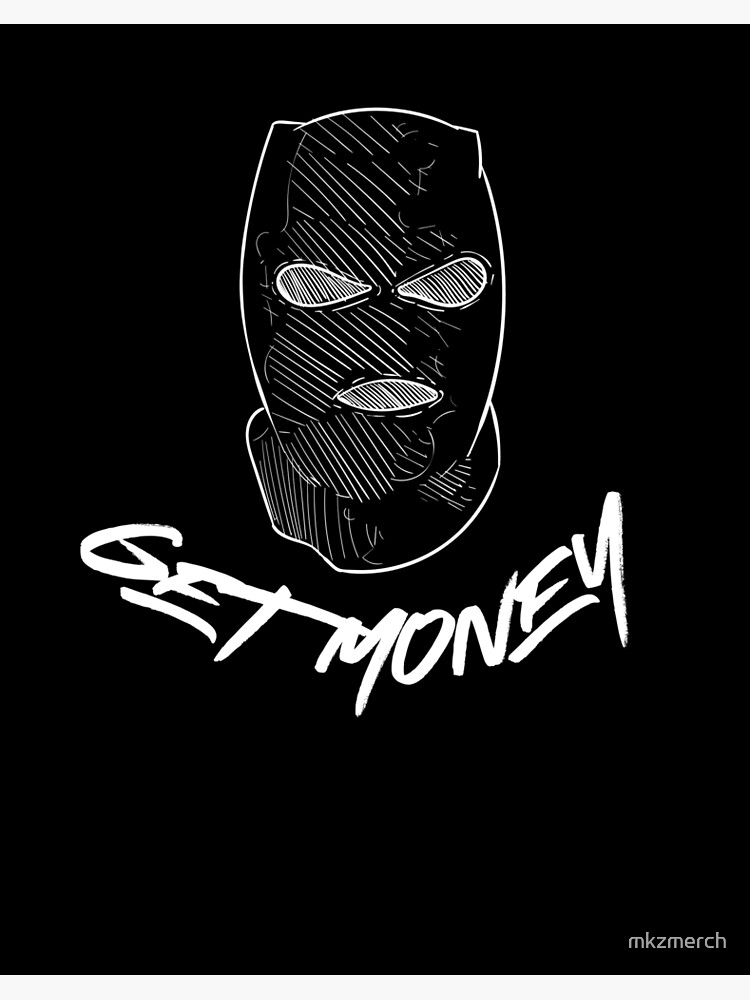The image is a vertically-oriented rectangular poster with a completely black background. Positioned centrally at the top is a black ski mask, detailed with a thin white outline to make it stand out. The mask features diagonal white brush strokes across it and includes oval-shaped eye and mouth holes that are marked with black and gray diagonal lines. Below the mask, in large, somewhat messy white text that curves downward in a semicircle, are the words "GET MONEY." In the bottom right-hand corner, there is small, light-gray text that reads "MKZ MERCH," likely indicating the creator of the poster.